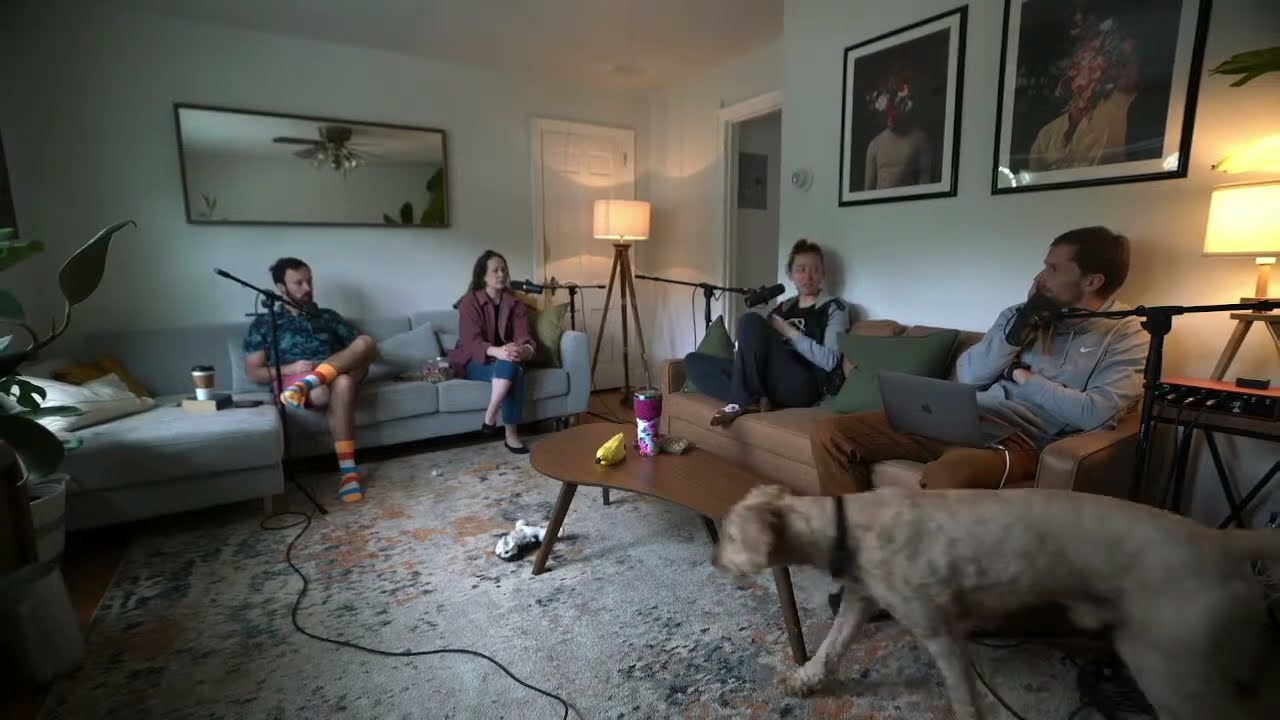In this image, four individuals, two men and two women in their twenties, are engaged in an intense podcast conversation while sitting on two different couches. The room features white walls and a worn, oriental rug on the floor. The man on the brown leather couch to the right wears brown pants, a gray shirt, and has a laptop in his lap, while the woman beside him appears in gray pants and a green shirt. In the background to the left, a man in a blue shirt with striped socks and a woman in a pink jacket and jeans sit on a gray couch. All four individuals have microphones in front of their faces. A tan, short-haired dog walks into the scene in the lower right corner. The setup includes a brown wood coffee table before the brown leather couch, posters, and a large mirror on the walls, suggesting a casual yet focused environment perfect for podcasting.